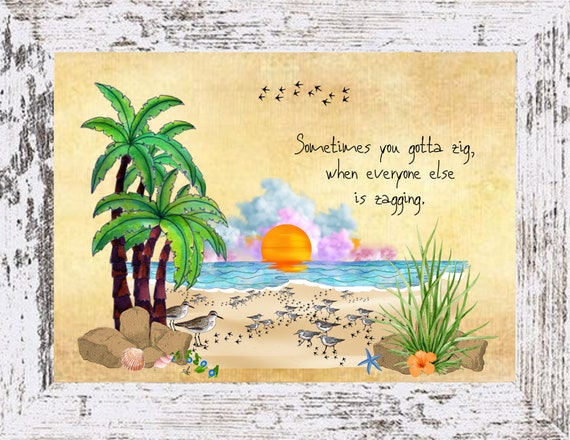This image captures a detailed watercolor beach scene framed by a distressed, wide wooden frame painted white with visible wear and tear. Dominating the left side of the painting are several tall palm trees and tan rocks, with a couple of small birds nestled beneath them. Scattered across the sandy beach are numerous smaller seagulls, their footprints intricately marked in the sand. Interspersed amid the birds are a few seashells. 

Transitioning towards the right, a lush, bush-like plant with a vibrant orange flower stands tall, accompanied by a blue starfish positioned nearby. The background features the serene light blue hues of an ocean, where the sun sits on the horizon, casting a bright orange glow. Puffy clouds in soft blue and pink hues drift above the sun, adding depth to the sky.

Near the top of the image, two lines of birds fly in silhouette. Embroidered across the scene is the motivational text, "sometimes you gotta zig even when everyone else is zagging," subtly blending into the dynamic elements of the artwork.